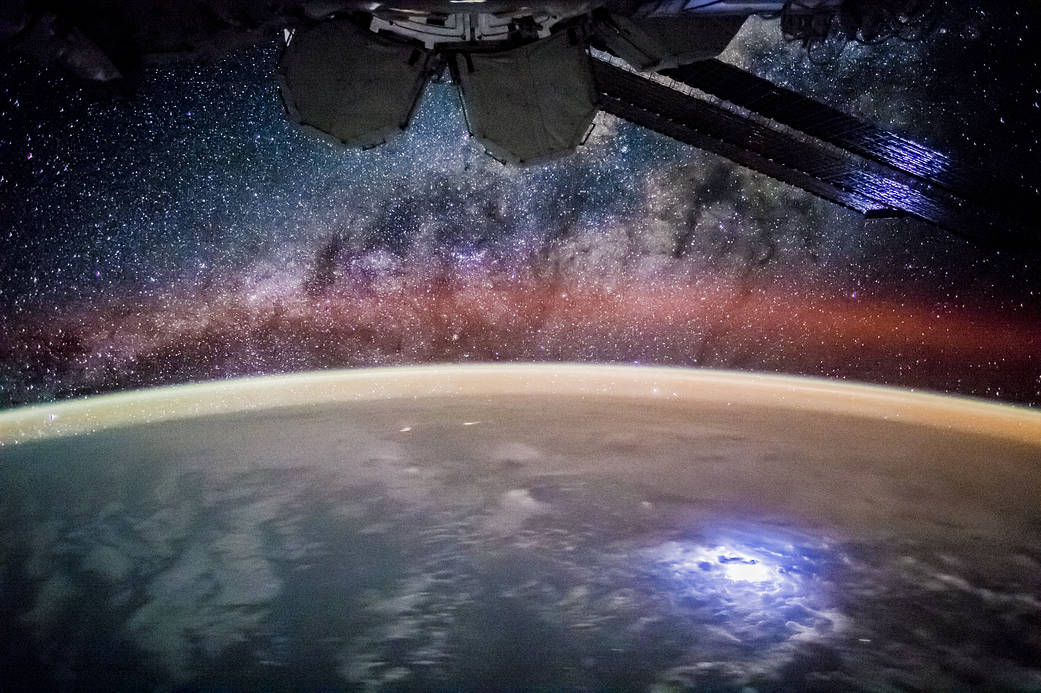The image captures a detailed view of planet Earth from space. The planet occupies the lower third of the image, displaying visible bodies of water, diverse landforms, swirling clouds, and a faint atmospheric edge. At the top of the image, a large satellite or space vehicle dominates the scene, positioned centrally and extending towards the right-hand side. The vehicle, which has a computer-generated appearance, is characterized by its black extended rods or antennas and capsule-like pods, emitting a blue glow from its right side. Reflections of this blue light are visible on the Earth's surface beneath the satellite. The star-filled sky in the upper third of the image is vividly illuminated with reds, purples, blues, and whites, contrasting with the dark, infinite space. The Earth, displaying a distinctive yellow border with brown and orange hues within, presents a striking semi-circular arc, lending a sense of depth and curvature. Overall, the scene is devoid of any people or text, providing a pure visual exploration of space and Earth’s celestial beauty.